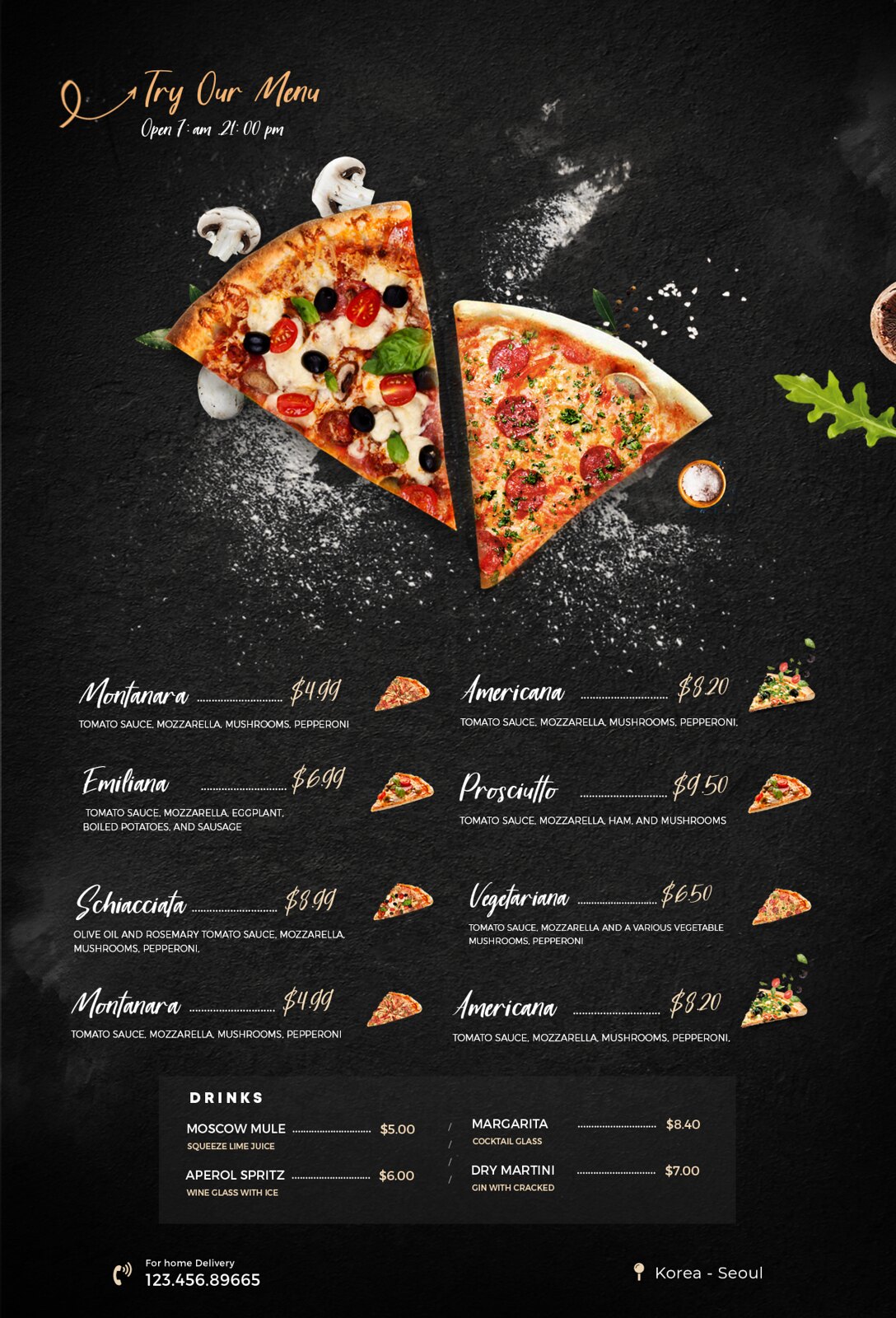Here is your detailed and cleaned-up caption:

"This is an image of a pizza menu set against a black background. In the top left corner, there is a playful squiggly arrow pointing towards a text that reads, 'Try Our Menu.' Below this, in very small text, the menu indicates the operating hours as 'Open 7 a.m. - 21 p.m.' Beneath this information are images of two large pizza slices. The slice on the left is topped with cheese, cherry tomatoes, what appears to be lettuce, and black olives. The slice on the right features cheese, pepperoni, and a sprinkling of a green herb. Adorning the background are flour and mushrooms, adding a rustic touch.

Below these pictures are the names and prices of various pizzas, each accompanied by a brief description of the ingredients and a corresponding image:
- Montanera: $4.99
- Americana: $8.20
- Emiliana: $6.99
- Prosciutto: $9.50
- Sciata: $8.99
- Vegetariana: $6.50
- Montanera: $4.99 (repeated)
- Americana: $8.20 (repeated)

Further down, the drink menu lists the following options:
- Moscow Mule: $5
- Margarita: $8.40
- Aperol Spritz: $6
- Dry Martini: $7

In the bottom left corner, there is a phone icon next to the text, 'For home delivery: 1-2-3-4-5-6-8-9-6-6-5.' In the bottom right corner, the location is marked as 'Korea, Seoul.'"

This detailed caption provides a clear overview of the pizza menu, including its design, specific items, and additional information about delivery and location.